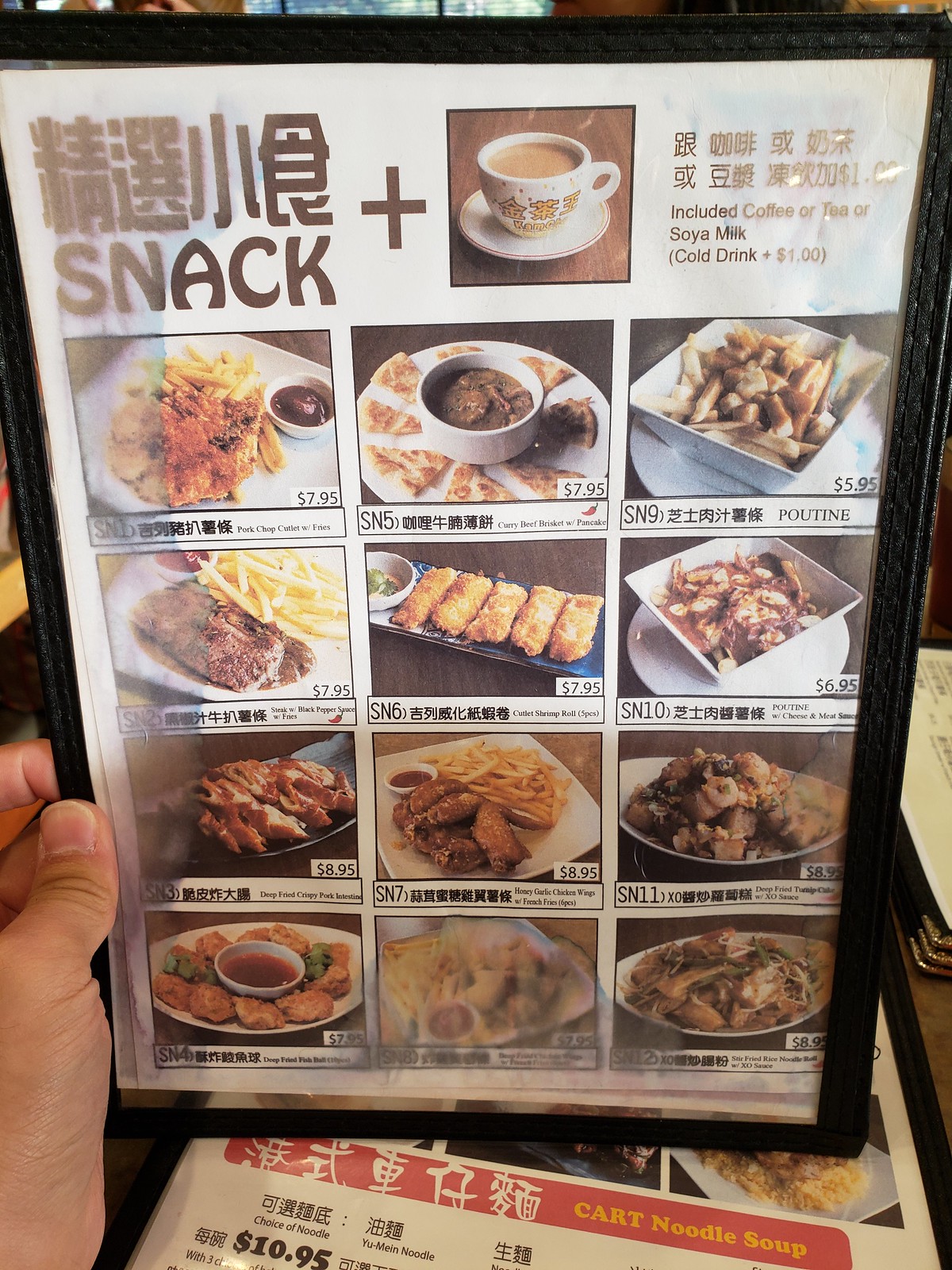A human hand is holding up a single-page menu from an Asian restaurant, featuring both Asian characters and English descriptions. At the top, there's a section labeled "Snack" with a plus sign and an illustration of a mug of coffee. On the right, it mentions that a coffee, tea, or soya milk is included. The menu displays around 12 different items with very small text, offering a variety of typical Asian dishes, including an unexpected poutine option. Beside it, flat on the table, another menu lists "Cart Noodle Soup" with a choice of noodles priced at $10.95.